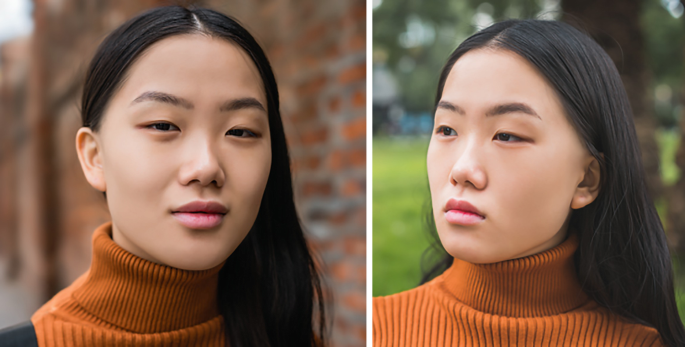This image features a young woman, likely in her early 20s, depicted in a photo grid comprising two side-by-side photographs. She has dark brown hair with a center parting, cascading smoothly behind her neck, and a flawless complexion that highlights her natural beauty. Her makeup is minimal, accentuating her plump, soft pink lips. In both photos, she wears the same copper-colored turtleneck, and the composition is cut off just below her neck.

In the left photo, she has a slight, almost imperceptible smile on her face, with her head tilted slightly to the right as she faces the camera. Her hair flows elegantly to her left shoulder. The background features a mix of blue and brown hues.

In the right photo, she appears more serious and contemplative, tilting her head slightly to the left while gazing off into the distance. Her hair remains parted in the middle but is styled to fall behind her neck. The background here transitions into blue and green tones, possibly suggesting a park-like setting. Her dark brown eyes and finely shaped eyebrows add to the depth and expressiveness captured in both portraits.